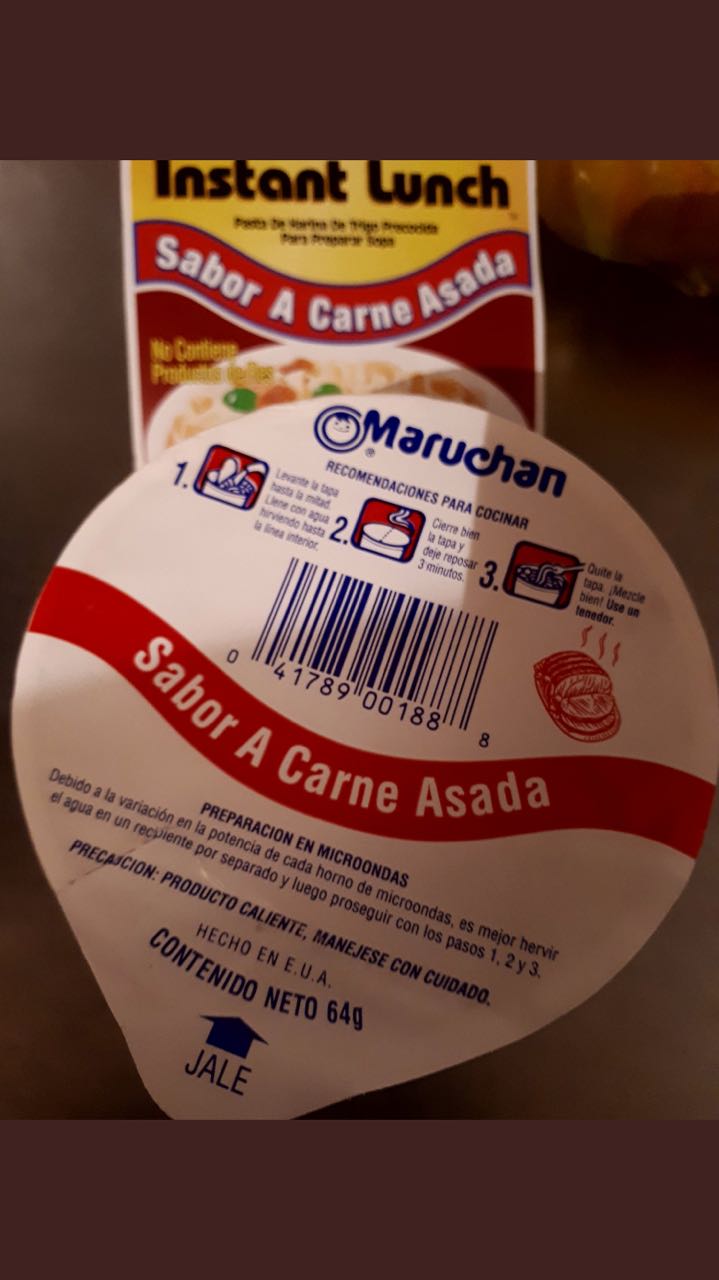The image showcases the top of a round package of instant ramen noodles, specifically a product by Maruchan. The package, which is slightly pointed at the lower left side, features a prominent red banner curved in the middle displaying the text "Seibor Akane Asada." The banner sits against a white background. At the top of the label, the brand name "Maruchan" is printed in bold blue letters. Beneath this, there are three distinct panels offering instructions for preparing the noodles. The center front of the label houses a barcode, adjacent to which is an image that appears to depict sliced meat. Additionally, preparation instructions in Spanish are located beneath the red banner. In the background, there is another package, predominantly yellow, white, and red, which displays a photograph of the prepared noodles and features the text "Instant Lunch" at the top in black letters.